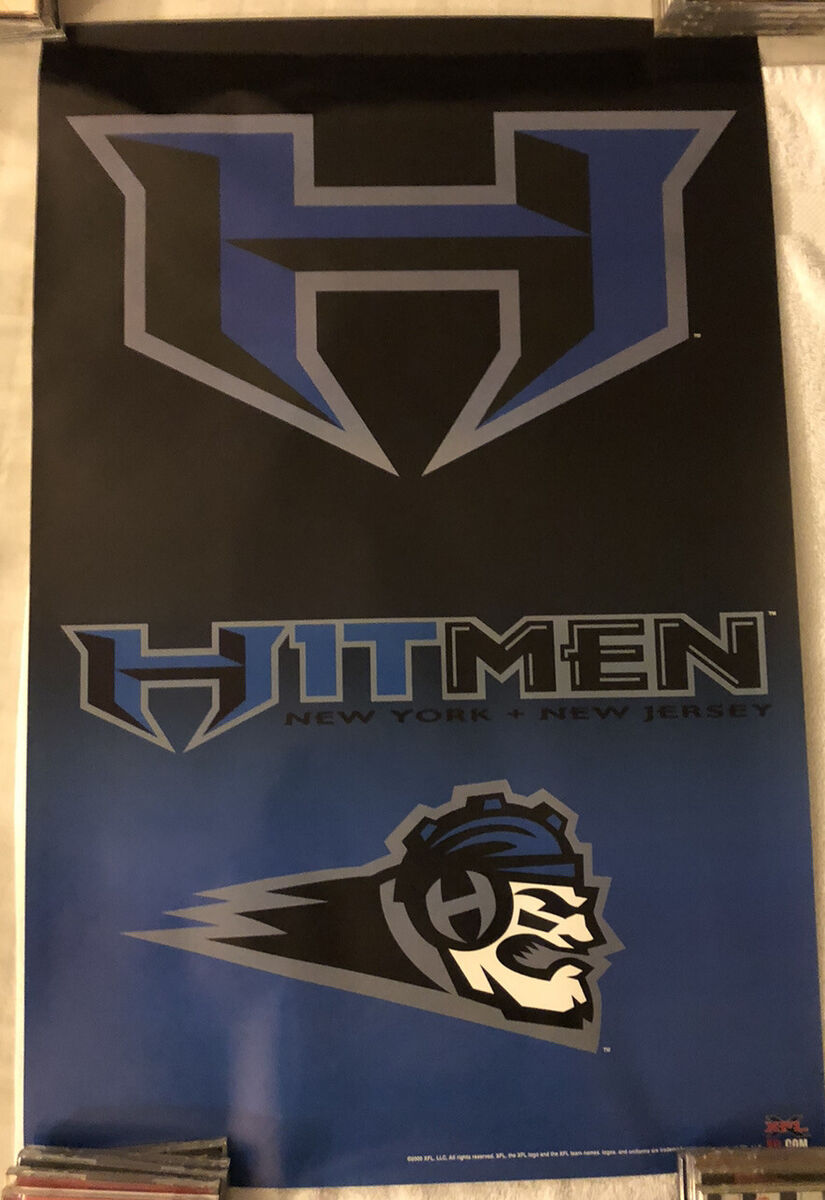The photograph captures a poster hanging on a yellowish surface, with a black and blue color scheme. Dominating the top portion of the poster is a stylized, 3D H-shaped logo that features a gray border and a mix of blue and black colors. The H has pointed ends, giving it a spiky appearance, and exhibits shadow effects for a 3D look.

Centering the poster is the title "Hitman," with "Hit" in blue and "Men" in black, accompanied by white outlines. Directly below the title, the words "New York" and "New Jersey" are printed in black font. Below this text is an illustration of an angry man’s white face, adorned with a blue and black helmet. His helmet and face are detailed, showing three rectangular attachments and a headset around his ears. 

Additionally, a pile of books occupies the bottom section of the poster, alongside more small white text. An object resembling a miniature house is placed in the bottom right corner of the image, enhancing the detailed scene. The background of the poster transitions smoothly from black at the top to navy blue at the bottom.